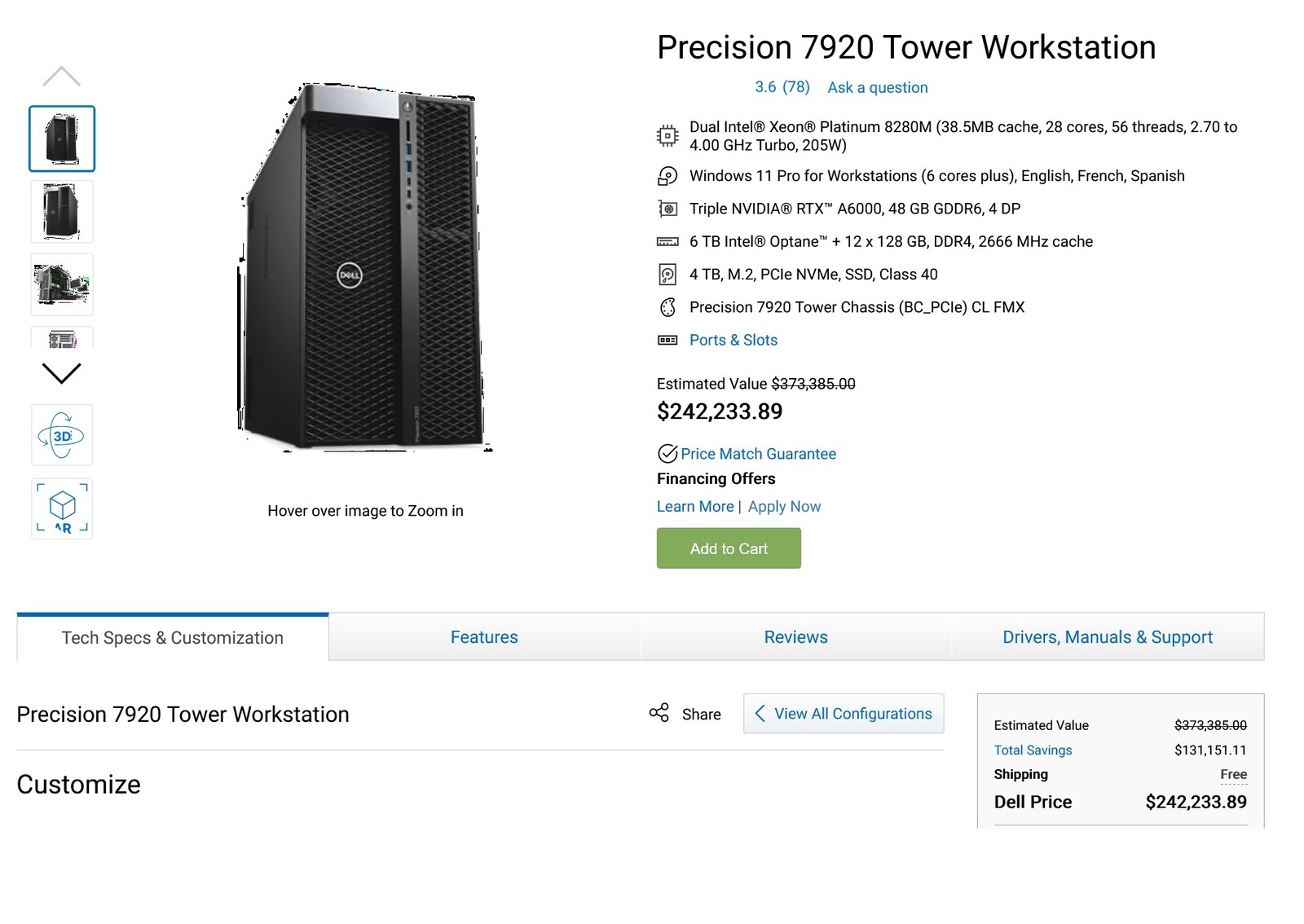This image depicts a detailed product page for the Dell Precision 7920 Tower Workstation. The central focal point is the workstation's tower, which is prominently displayed in sleek black. Various thumbnail images of the device are aligned in a vertical column on the left side of the image, allowing for different viewing angles and close-ups when clicked. 

The Dell logo is clearly visible on the front of the tower, which is notably larger than a typical desktop computer tower. The image includes a hover-over feature for zooming in on specific parts of the workstation. 

On the right side, detailed specifications are provided. The Precision 7920 Tower is reviewed 78 times with an average rating of 3.6 stars. Detailed descriptions include dual Intel Xeon Platinum processors, Windows 11 operating system, triple NVIDIA RTX graphics cards, a 6-terabyte Intel Optane storage module, and a 4-terabyte M.2 Class 40 drive. Additional information about ports and slots is available as well. 

The total estimated value of the workstation is listed at $242,233.89, with financing options available via a provided link. The page also highlights various tabs for technical specifications, customization options, features, reviews, drivers, and current savings, which indicate a significant reduction from its original estimated value of over $300,000.